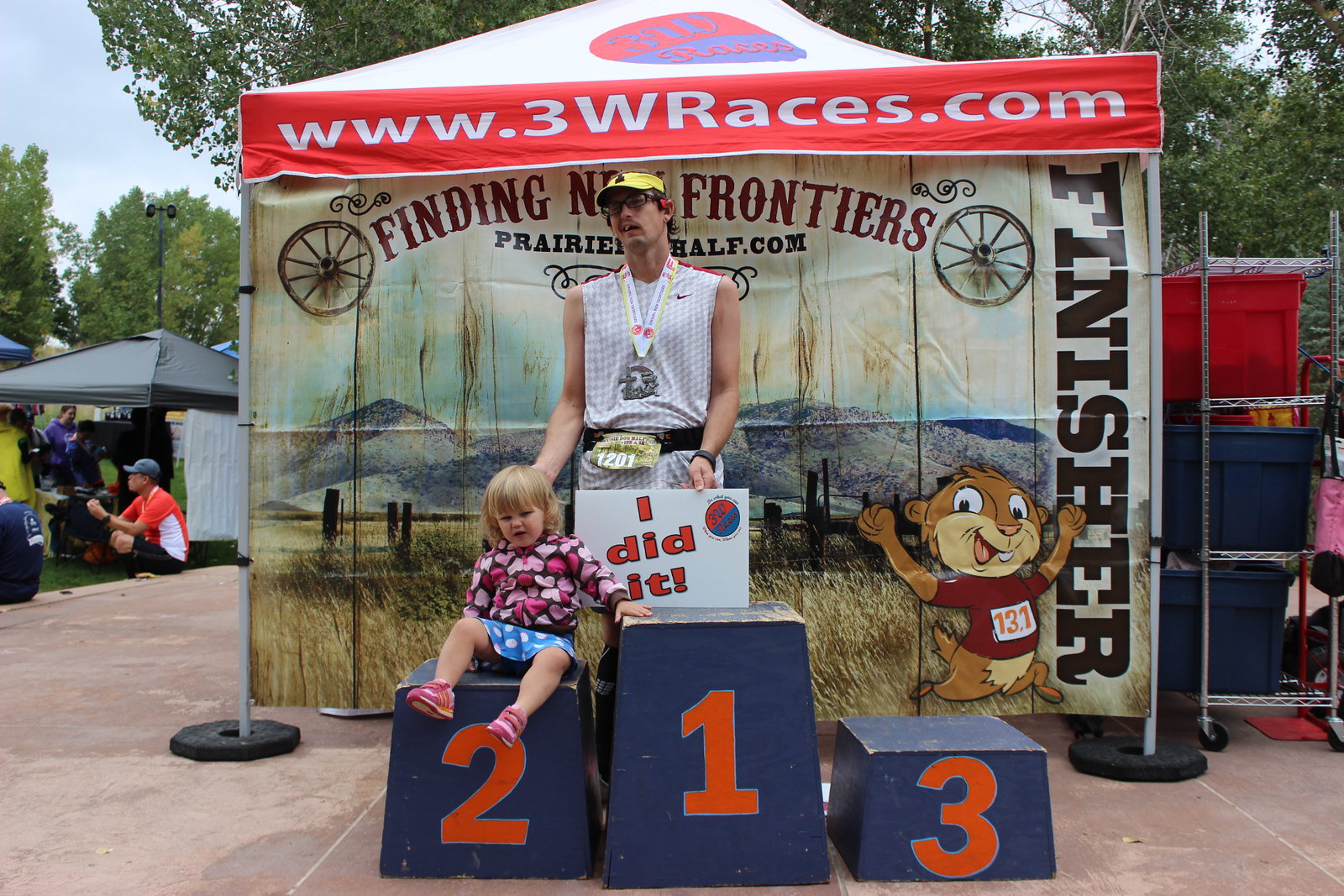This photograph captures a celebratory moment at a race finish line. Central to the image is a winner's podium composed of three blue-painted wooden pedestals marked with red numbers. The tallest, positioned at the center, displays a "1," the second tallest on the left shows a "2," and the shortest on the right has a "3." Seated on the number two pedestal is a small child adorned in a blue skirt with white dots, pink shoes, and a long-sleeved jacket decorated with pink hearts. 

Behind the podium, a man, presumably the child's father, stands proudly. He wears a sleeveless tan and white-striped plaid shirt, a yellow visor, dark sunglasses, and a thick necklace. A racing ticket with the number 1201 is secured around his waist, while he holds up a white sign boasting "I did it!" in red letters. Further identification details include a metal around his neck, highlighting his race participation.

The background reveals a tent with a banner displaying the website www.3wraces.com. Adjacent signage reads "Finding New Frontiers prairiehalf.com" with the word "Finishers" indicating this is the race's conclusion point. The scene is bustling with other people and booths, including a visible man wearing a red shirt sitting among the crowd and distant trees completing the backdrop.